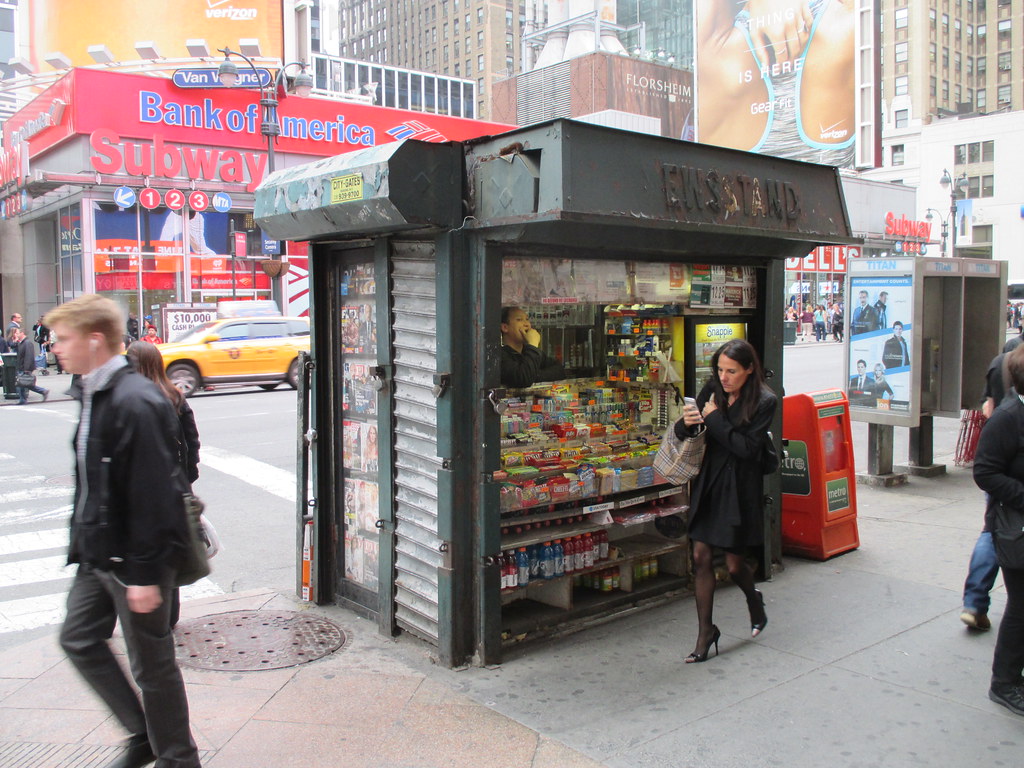The image is a vibrant color photograph capturing a bustling city street, likely in New York, centered around a busy newsstand. Positioned on a concrete sidewalk at a street corner, the newsstand has a black metal exterior and a rolling gate visible on the left, with magazines displayed behind glass. The front is wide open, showcasing shelves filled with candy and drinks, and a cooler labeled Snapple. An orange newspaper dispenser with "Metro" in white text on a green background is situated to the right of the newsstand. 

A man, appearing to be of Asian descent and wearing a long-sleeved black shirt, stands behind the counter, his elbow resting on a shelf filled with candy and his hand thoughtfully positioned on his chin. To the right of the stand, there is also a telephone booth. 

In the background, tall skyscrapers with advertising billboards dominate the skyline. The street scene includes a yellow taxi cab and numerous pedestrians on the sidewalk, including a woman in high heels engrossed in her phone. Prominent landmarks include a Bank of America branch adorned with blue text and a red "Subway" sign indicating the 1, 2, and 3 subway lines. Additional details like a crosswalk, a manhole cover, and the lively movement of people underscore the dynamic atmosphere of the city.